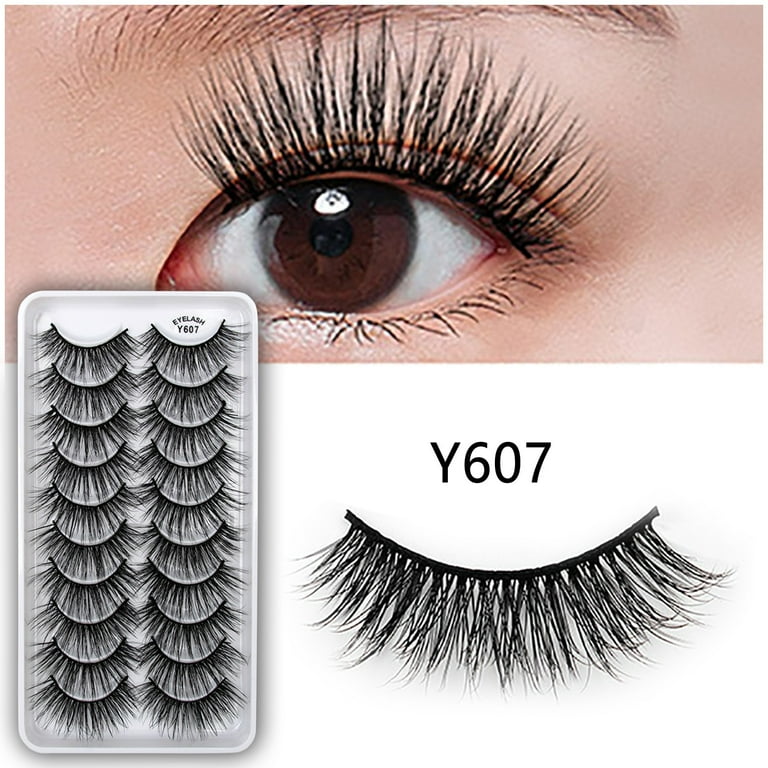This advertisement image, ideal for online marketplaces like Amazon or eBay, features a detailed close-up of a brown Asian eye adorned with lush, long false upper eyelashes, complemented by shorter lower lashes. The bottom portion of the brown eyebrow is also visible. Below and slightly overlapping this eye image is a white rectangular tray filled with 20 false eyelashes, organized into two vertical rows of 10. The tray prominently displays the label "Y607." To the lower right of the image, against a white background, the label "Y607" appears again in large black text, accompanied by an enlarged view of one of the false eyelashes.